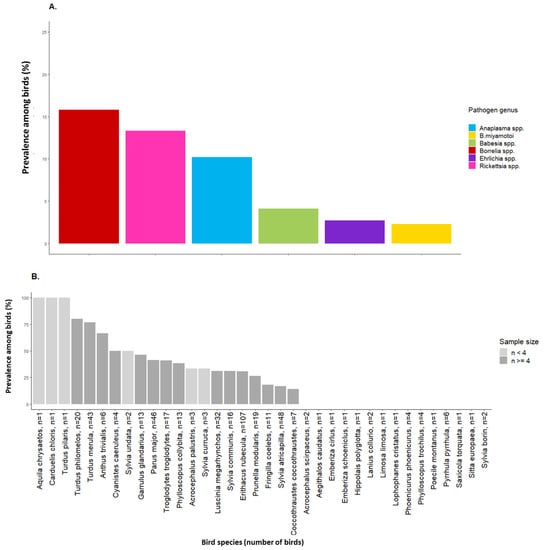The image displays two bar graphs, labeled A and B. Bar graph A features a colored bar representation illustrating the prevalence of various pathogens among bird species, with the y-axis labeled as "Prevalence among Birds (%)". The bars are color-coded as follows: red for B. bohelia, blue for anaplasma, pink for R. rickettsia, yellow for B. malleable, green for B. albisa, and purple for E. ecria. Graph B, presented in gray bars, shows the sample sizes of bird species, with the x-axis labeled "Bird Species Number of Births", ranging from N1 to N48. This graph indicates the number of birds sampled, with some species having bars representing their sample sizes while others do not. Both graphs are aligned with the purpose of illustrating and comparing the prevalence of pathogens and the bird species sample sizes.